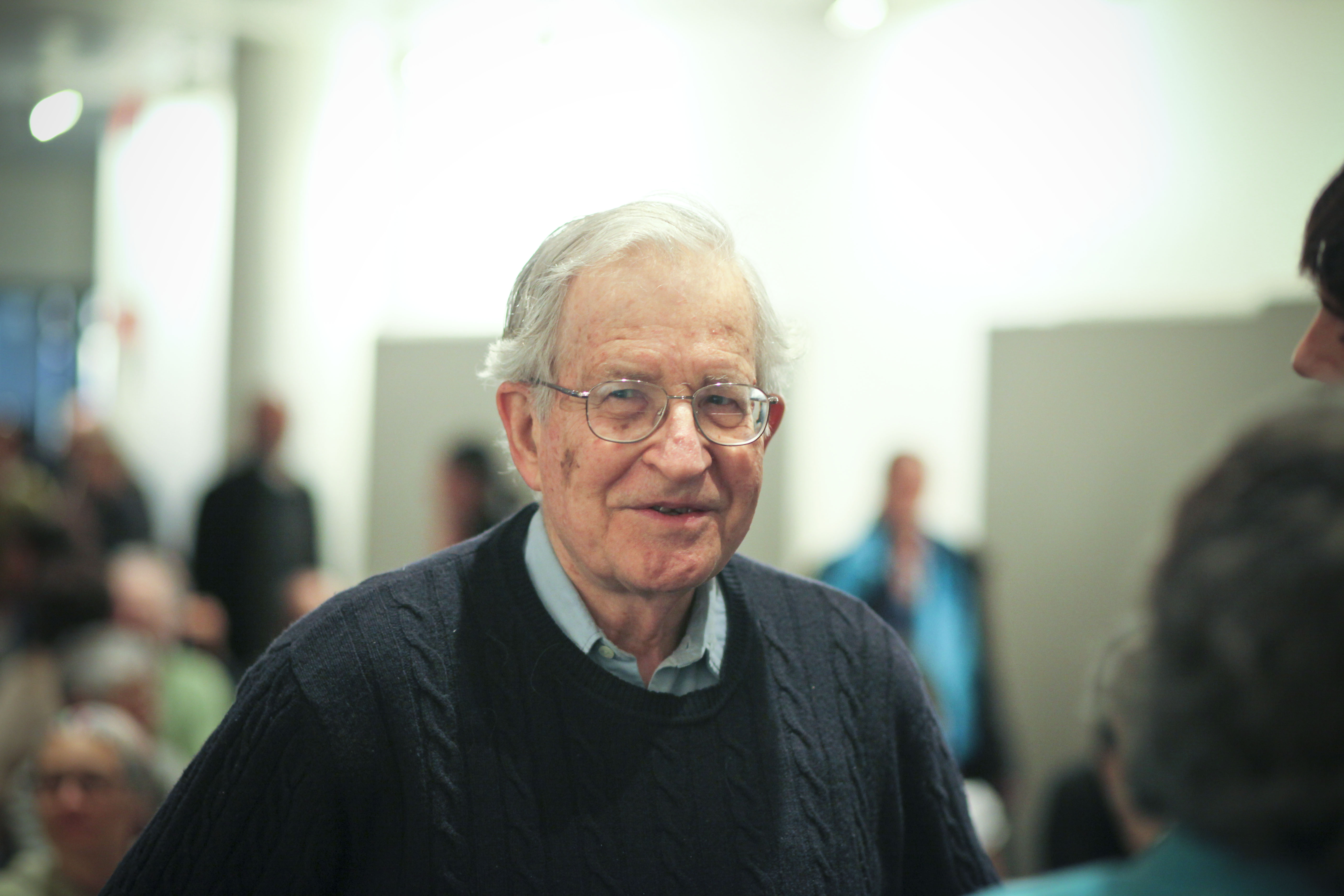In the image, an elderly man is prominently placed in the center, facing the camera while glancing to the left. He wears wire-framed glasses, a soft smile, and a blue cable-knit sweater over a light blue collared shirt. The background, though blurred, reveals a busy indoor setting that resembles a senior center, with several individuals discernible but not in focus. The walls are white, and various bits of furniture and lights create an inviting ambiance. Just to the right of the elderly man, there is an out-of-focus individual with gray hair and a blue garment, and another person partially visible. The overall colors include black, light blue, tan, gray, green, and white, contributing to a daytime indoor scene.